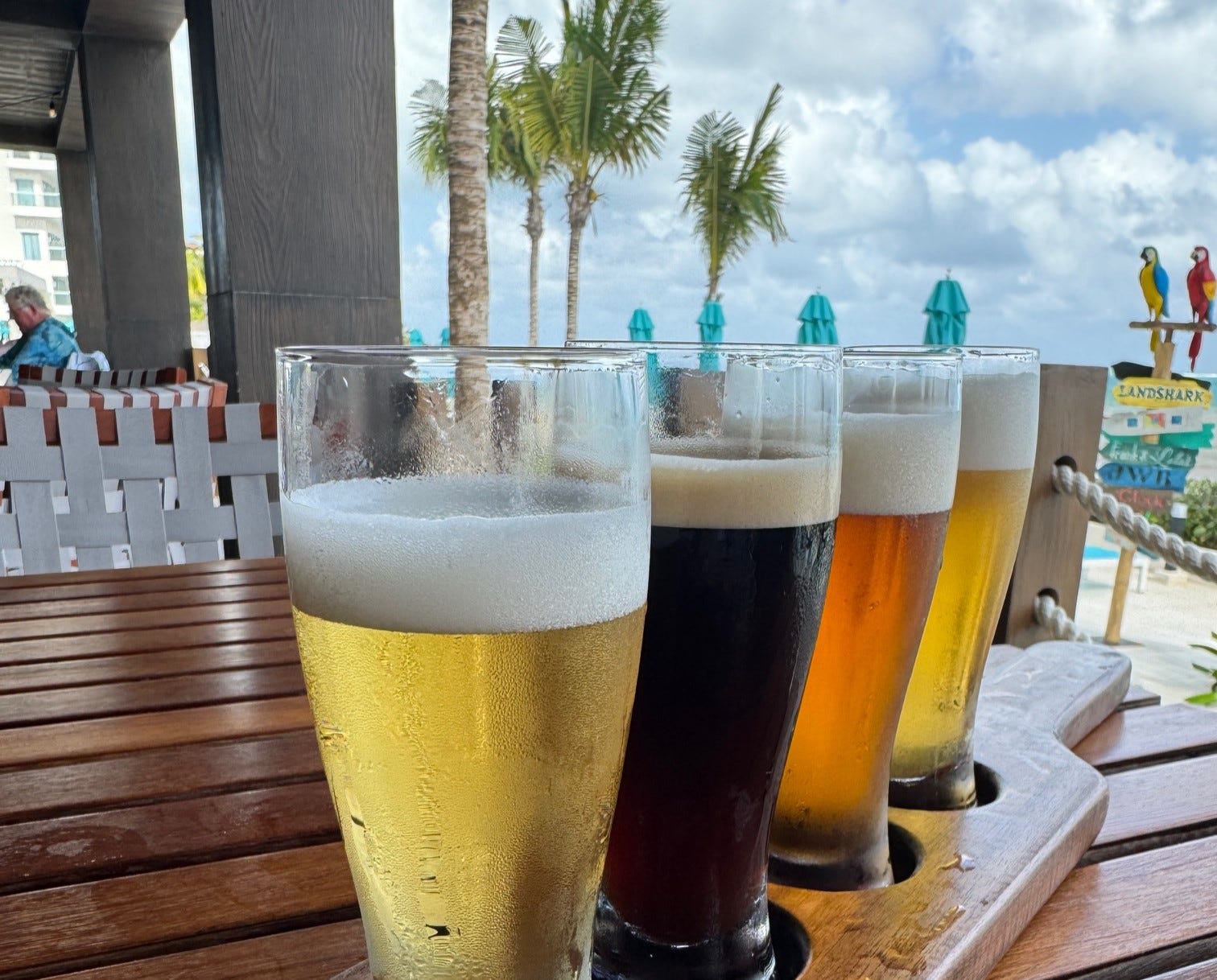In this vibrant beachside scene, an outdoor pub with a relaxed lounge atmosphere is captured in a photograph. At the forefront is a wooden table with dark-stained wood slats, showcasing a flight of four beer varieties, each in glasses that seem pint-sized. The beers are carefully arranged in a wooden paddle with round cut-outs for the glasses. The first beer, on the far left, is a clear, golden blonde with a white foamy top. Next is a deeper, chocolate-colored stout with a creamy foam head. The third beer presents an amber hue, while the fourth glass holds a dense, golden brew. In the background, a lively dining area is visible, featuring a white fence, tables with older patrons, and sturdy, gray pillars. The setting is adorned with numerous palm trees and vibrant, teal umbrellas, under a bright blue sky with scattered clouds. A sign on the right side reads "Landshark," and nearby are two colorful parrots, enhancing the tropical ambiance.